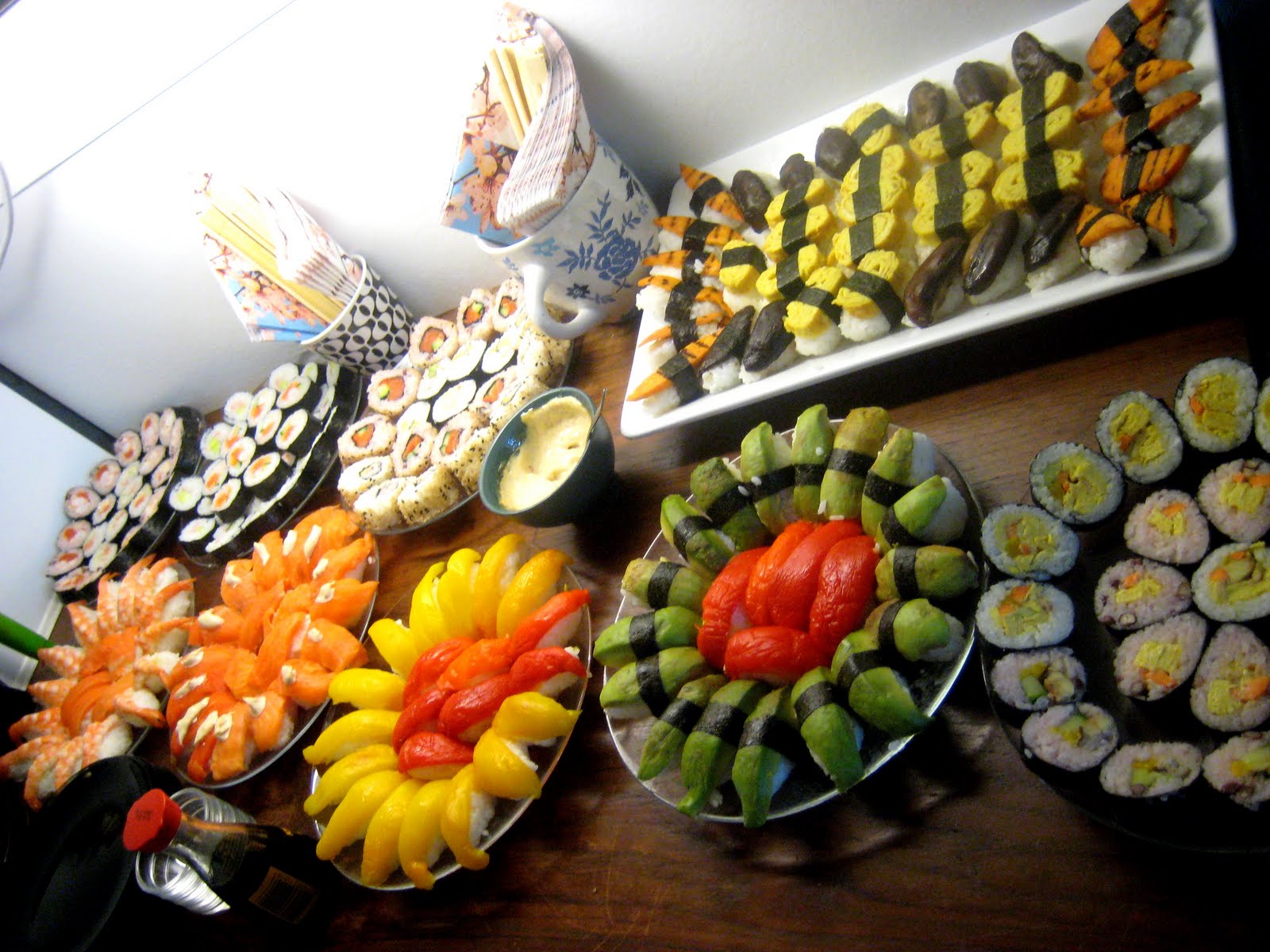This vibrant color photograph, taken from a unique angle, captures an elaborate spread of sushi on a long, dark hardwood table. The perspective creatively distorts the image, making the table appear as though it is a vertical surface. However, it is unmistakable that this is a table due to the delectable selection of sushi artfully arranged on it.

In the foreground, several large, round plates showcase a variety of sushi. California rolls and sashimi, with their strikingly beautiful orange hue, dominate the scene. Particularly eye-catching is a sushi arrangement featuring pieces with a bright yellow color, meticulously placed to resemble the petals of a flower. Additionally, there is another set of sashimi in a darker shade of orange, adding a diverse color palette to the display.

On the upper right-hand corner of the image, a long white tray holds an assortment of sushi rolls, further enriching the visual feast. The classic sushi rolls, wrapped in nori, are presented alongside the more artistic creations, making for an aesthetically pleasing and mouth-watering presentation.

This photograph not only highlights the culinary artistry of sushi but also leverages a distinctive camera angle to create the illusion that the sushi is adorning the wall, providing a surreal and captivating visual experience.